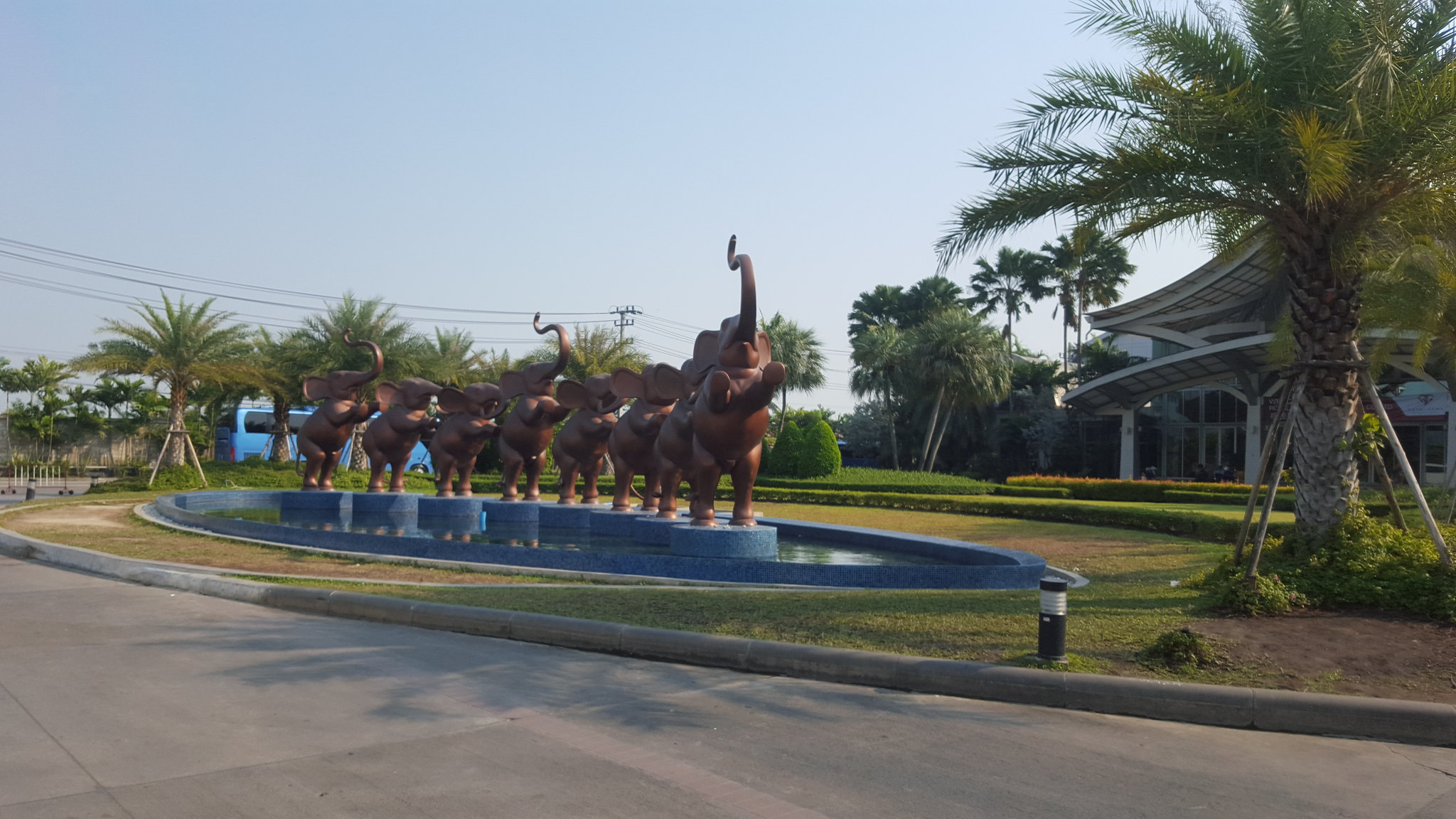This photograph captures a whimsical outdoor scene, likely located in a tropical region. The focal point is an oval-shaped fountain, paved in blue, situated within a circular driveway. The fountain features seven goldish-brown elephant statues standing on individual blue pedestals. Each elephant stands on its hind legs, with its front legs resting on the back of the elephant in front of it, forming a line. Most of the elephants have their trunks raised in the air. The fountain is surrounded by lush green grass and encircled by well-maintained hedges. To the right, there is a notable fat palm tree, among several other palm trees that are braced with supporting sticks. In the background, under a clear blue sky, stands a large, visually appealing building that could be a museum, a fancy resort, or a private residence. There's also a blue work van visible near the building. A concrete curb and a post with a light top off the detailed surroundings of this picturesque setting.